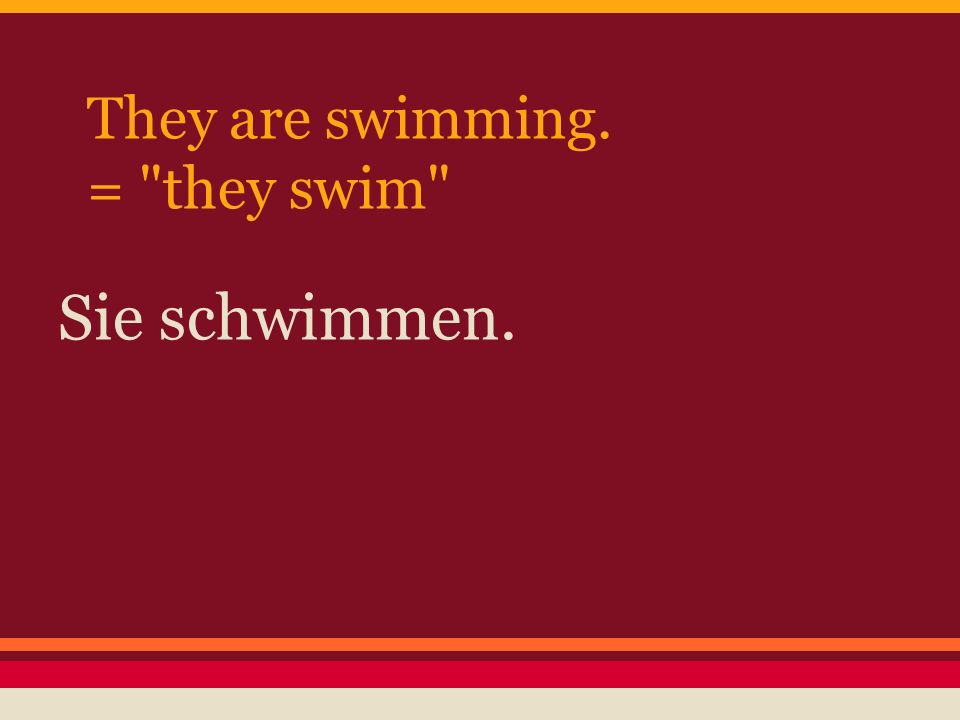This image appears to be an educational slide, likely created in PowerPoint, that aims to teach a phrase in German. The background is predominantly burgundy, with an arrangement of color stripes adding detail: a golden yellow stripe at the very top, followed by a narrow orange stripe, then a red stripe, and finally a beige stripe at the very bottom. The main section of the slide features three lines of text aligned to the left. The first line, in golden yellow Garamond font, reads "They are swimming." Directly below, the text "= 'They swim,'" also in golden yellow, explains the equivalent phrase. The third line of text in beige reads "Sie schwimmen," which is the German translation. The setting and style of this slide suggest it's part of an educational presentation, meant to instruct learners on how to convert an English phrase into German.